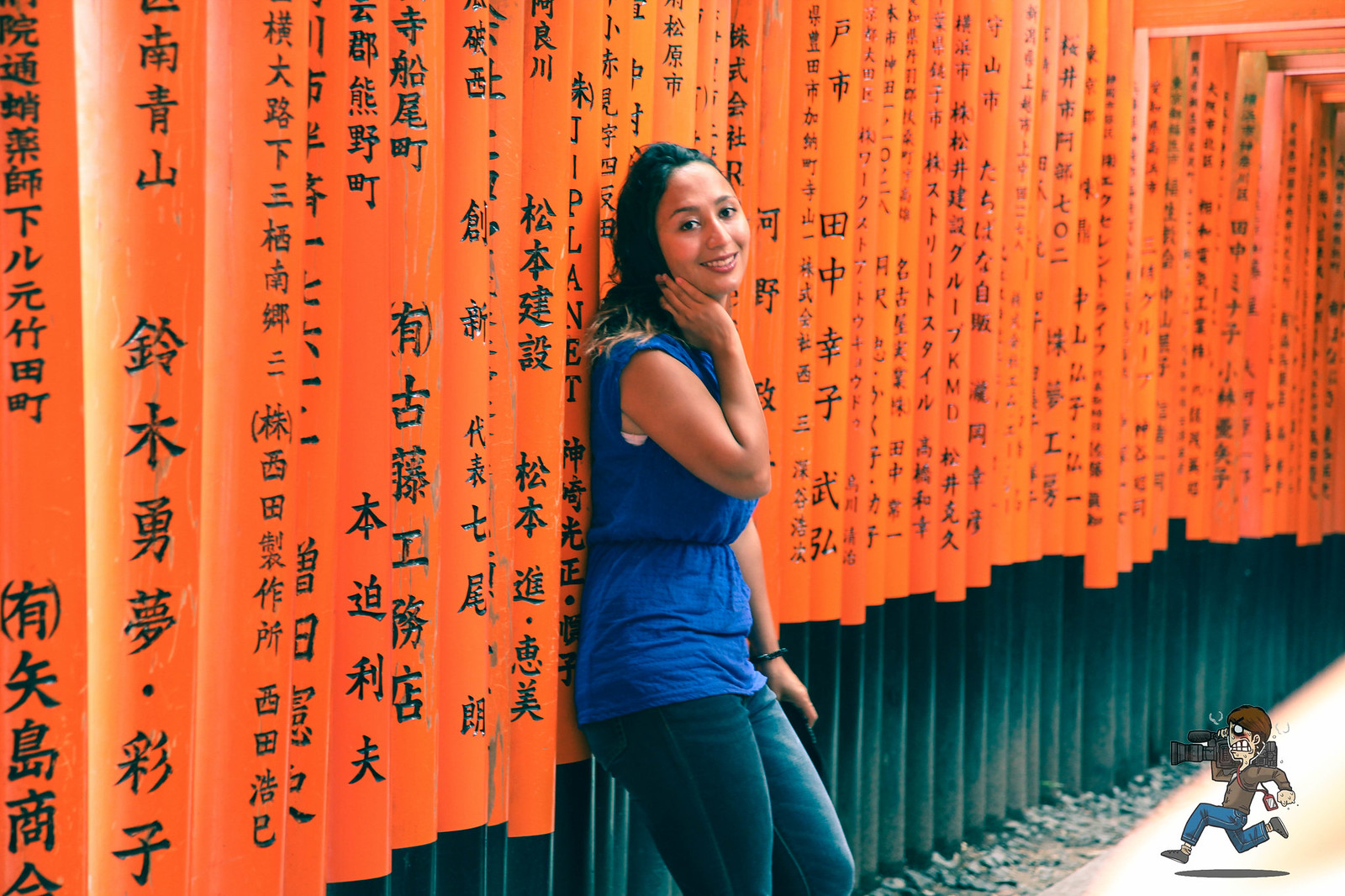A young woman, possibly of Indian descent, is leaning against the vibrant orange torii gates at the iconic Fushimi Inari Taisha Shinto shrine. She is dressed in a bright blue blouse with short sleeves and blue jeans. Her dark hair cascades down her shoulders as she smiles warmly at the camera, with her right hand bent under her chin. The torii gates display numerous Japanese symbols running vertically, and they transition to a dark green color about two feet from the ground, creating a striking contrast. The ground beneath her is scattered with rocks, and in the lower right corner of the image, a tiny cartoon depicting a running figure with scissors can be seen, adding an unexpected whimsical touch.